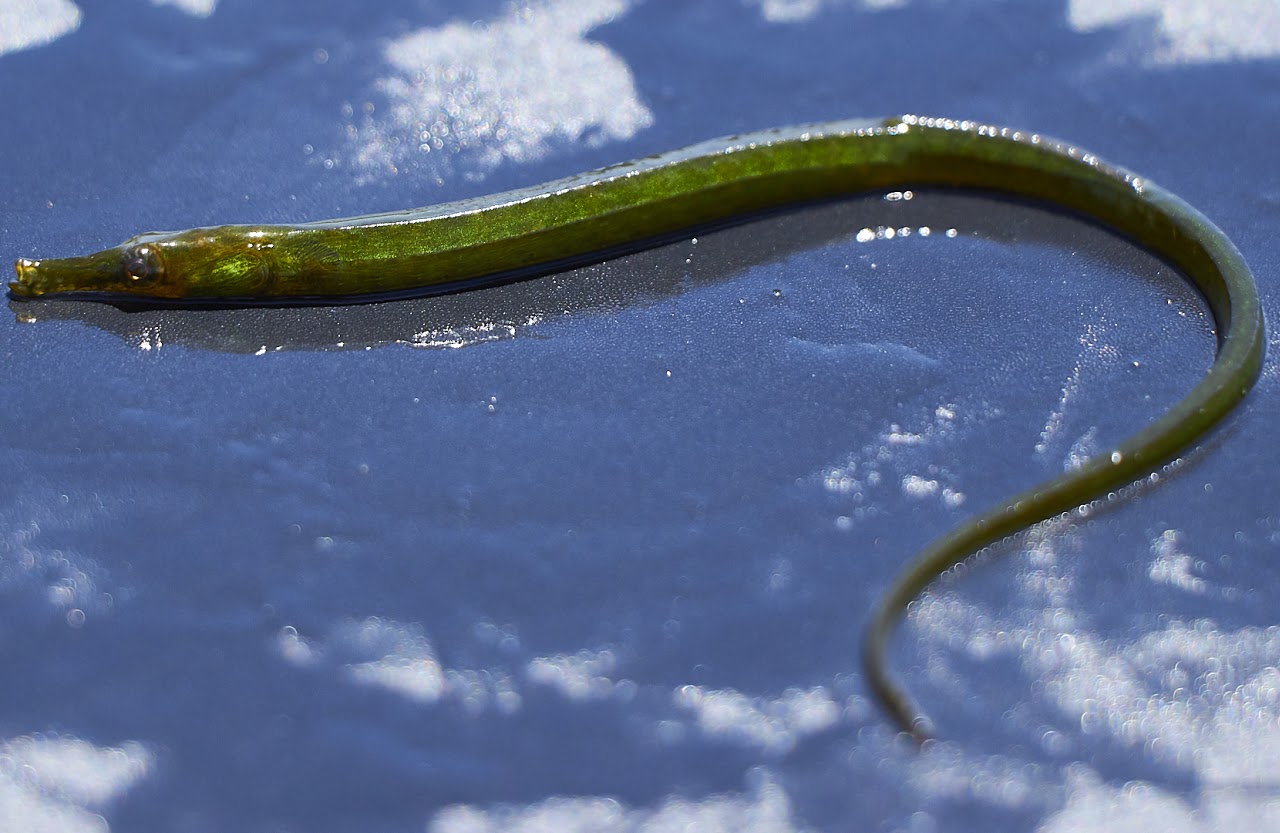In the detailed photograph, a long, green, slimy creature resembling a worm, eel, or leech is depicted on a wet, blue surface with light reflections. The creature, featuring a glossy, shiny, and water-repelling skin, has a body tapering towards the tail end. Its greenish color is interspersed with a bit of brown, especially around the head area. The head bears a resemblance to a seahorse's snout, with characteristics similar to a suction cup. The overall image has a zoomed-in perspective, where the creature appears to slither, hinting at possible ice chunks around it. A light source from the upper right highlights the wet surface, which could resemble sand or mud, adding to the glossy appearance of the creature.